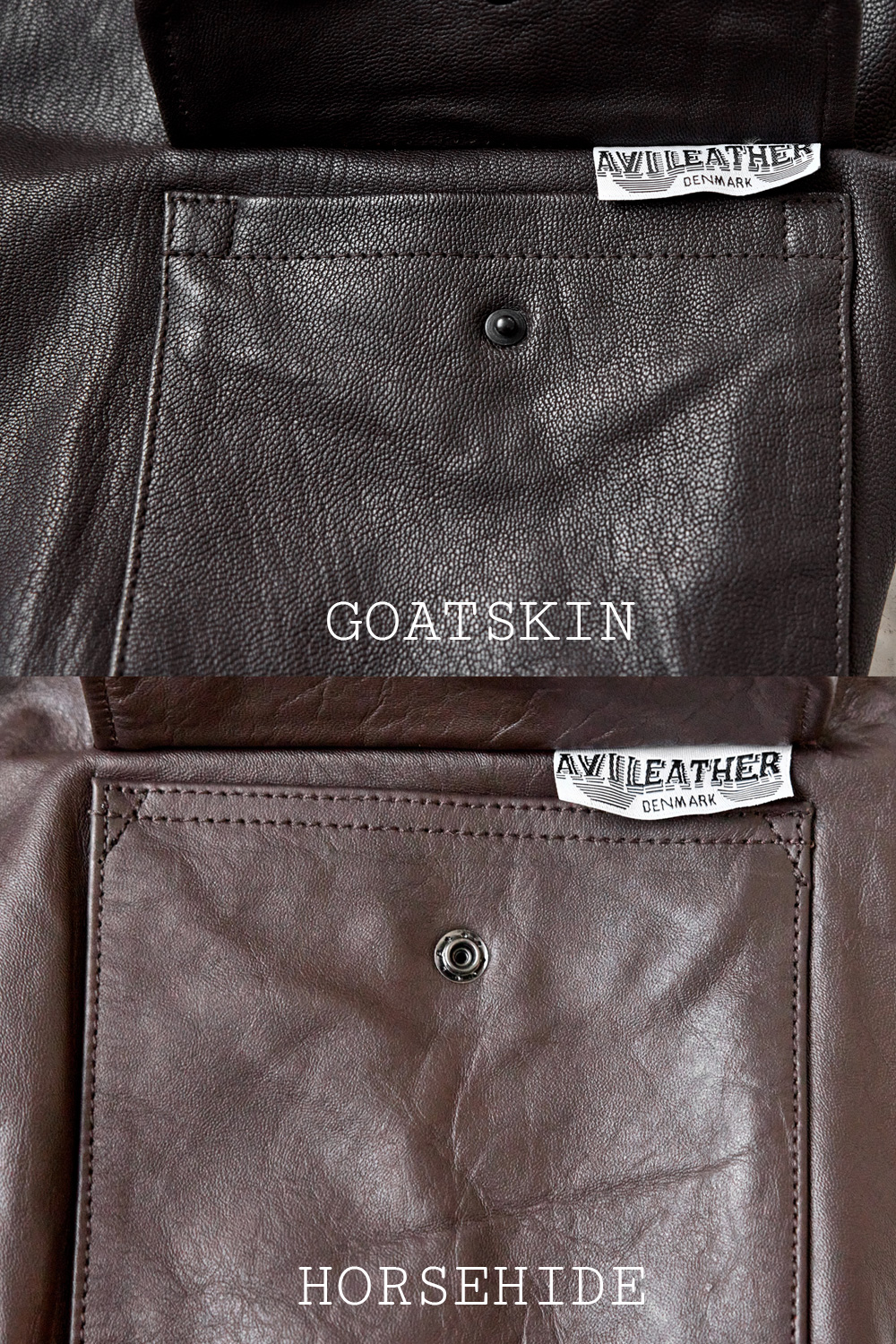This image is a collage of two detailed photographs showcasing different types of leather materials, presented as part of an advertisement for ABI Leather, a brand from Denmark. The image is evenly divided into two sections, each highlighting a different type of leather and a pocket.

The upper half features black goatskin leather with a fine pebbly texture. The pocket in this section is open, revealing meticulous stitching and a tag that reads "ABI Leather Denmark." Beneath the pocket, the leather is labeled "GOAT SKIN" in white capital letters.

The lower half displays dark brown horsehide leather, characterized by a smoother, slightly wrinkled texture. This section also includes an open pocket with a tag that reads "ABI Leather Denmark." A grayish-black metal snap is partially visible, suggesting the functionality of the pocket. The leather in this part is labeled "Horse Hide" in white text.

Both pockets share a consistent branding style with the ABI Leather Denmark tag and exhibit excellent craftsmanship, underscoring the high quality of the leather.